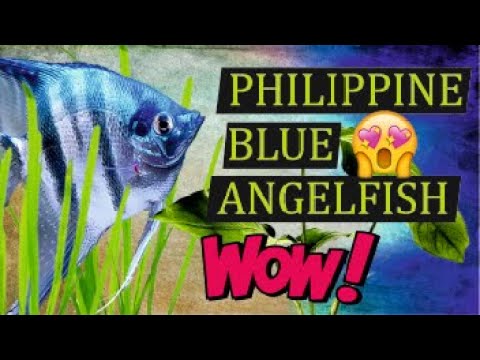The image appears to be a low-resolution, digital artwork or still frame from a video, likely designed as a poster or background for a computer or phone screen. It features a bluish-tinted Philippine blue angelfish, depicted in a tall, triangular shape, with its mouth pointed to the right. The angelfish is situated on the left side of the image, swimming amidst green plants, seagrass, or seaweed. On the right side, there are three black rectangles stacked vertically, each containing a line of yellow text that together read "Philippine blue angelfish." Additionally, there’s a comic book-style, red text with a black outline that exclaims "WOW!" This "WOW!" text is accompanied by an emoji with heart eyes, enhancing the sense of admiration and excitement conveyed by the image.